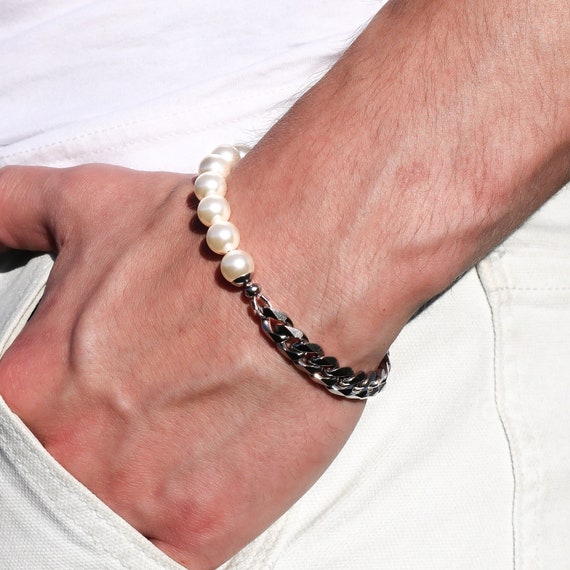The square photograph features a rather close-up image of a white person's hand partially extended into the pocket of white pants or shorts. The garment appears to be made from a heavy fabric with white stitching, complemented by a white t-shirt seen at the top of the hand. The skin is pinkish-white with visible veins and light hair on the forearm above the wrist. The hand, positioned facing down towards the bottom left corner, has its fingers inside the pocket while the thumb extends out, partially cut off at the edge of the image. The central focus is a beautiful bracelet on the wrist, combining a polished silver chain on the bottom half and what appears to be real pearls on the top half, connected by silver hardware. This intricate jewelry draws immediate attention, contrasting elegantly against the monochromatic clothing background.